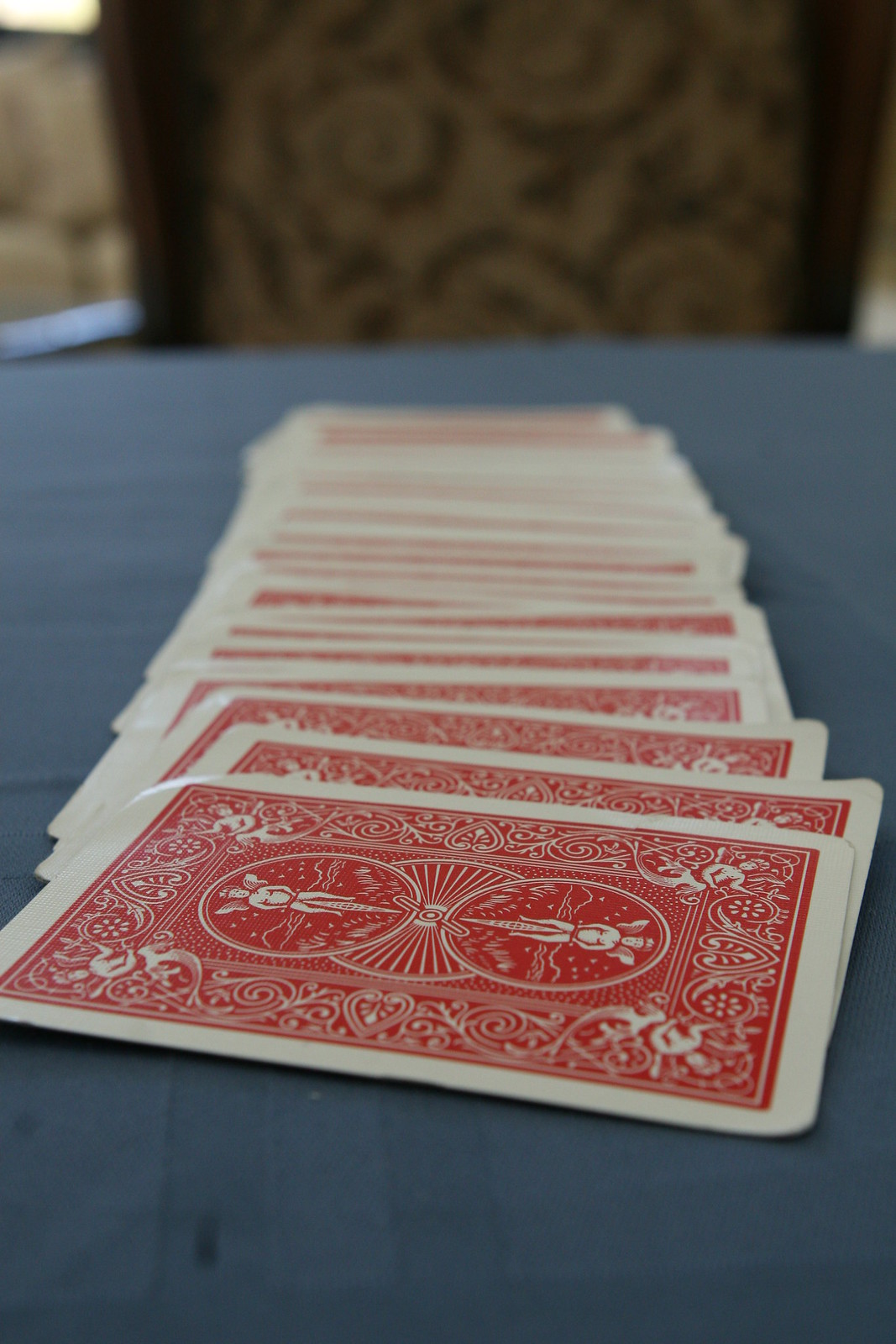A photograph captures a full deck of cards face down, meticulously spread out in a fan formation across a richly colored green or teal tablecloth. The card backs are adorned with a vibrant red design, each card featuring two circles enclosing cherubic figures—one cherub facing left, the other right, which would appear as up and down if the cards were oriented vertically. The sharp focus highlights the intricate details of the nearest cards, while the rest gradually fade into a soft blur. At the far end of the table, nestled slightly out of focus, stands an ornate wooden chair embellished with antique spiral upholstery—indicative of a dining room or vintage setting. The composition suggests a prelude to a captivating magic trick, hinting at the anticipation and mystery that lies just beyond the frame.